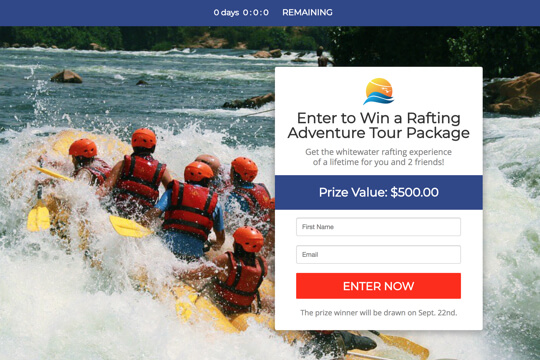The upper section of the page features a header with a dark blue background and centered white text that reads "00:00:00 REMAINING" in capital letters. The main part of the page has a background image of a group of people engaged in whitewater rafting. Each participant is outfitted in red life jackets with black straps and bright orange helmets adorned with black dots, except for one individual at the center-back who wears a beige or pinkish helmet. They are all in a yellow raft surrounded by crashing waves. The group holds a mix of paddles: some have long yellow poles with yellow blades, while others have black poles. In the distance, ripples of waves and several rocks jutting out of the water are visible.

On the right side of the page is a rectangular overlay with a white background, featuring clip art of the sun and waves. The sun is depicted as a simple circle with a gradient transitioning from yellow on the left to orange on the right, topped with a white curved line. Below the sun are thick, curvy blue lines representing waves. Beneath the clip art, black text invites viewers to "Enter to win a rafting adventure tour package," with smaller gray text underneath adding, "Get the whitewater rafting experience of a lifetime for you and two friends!"